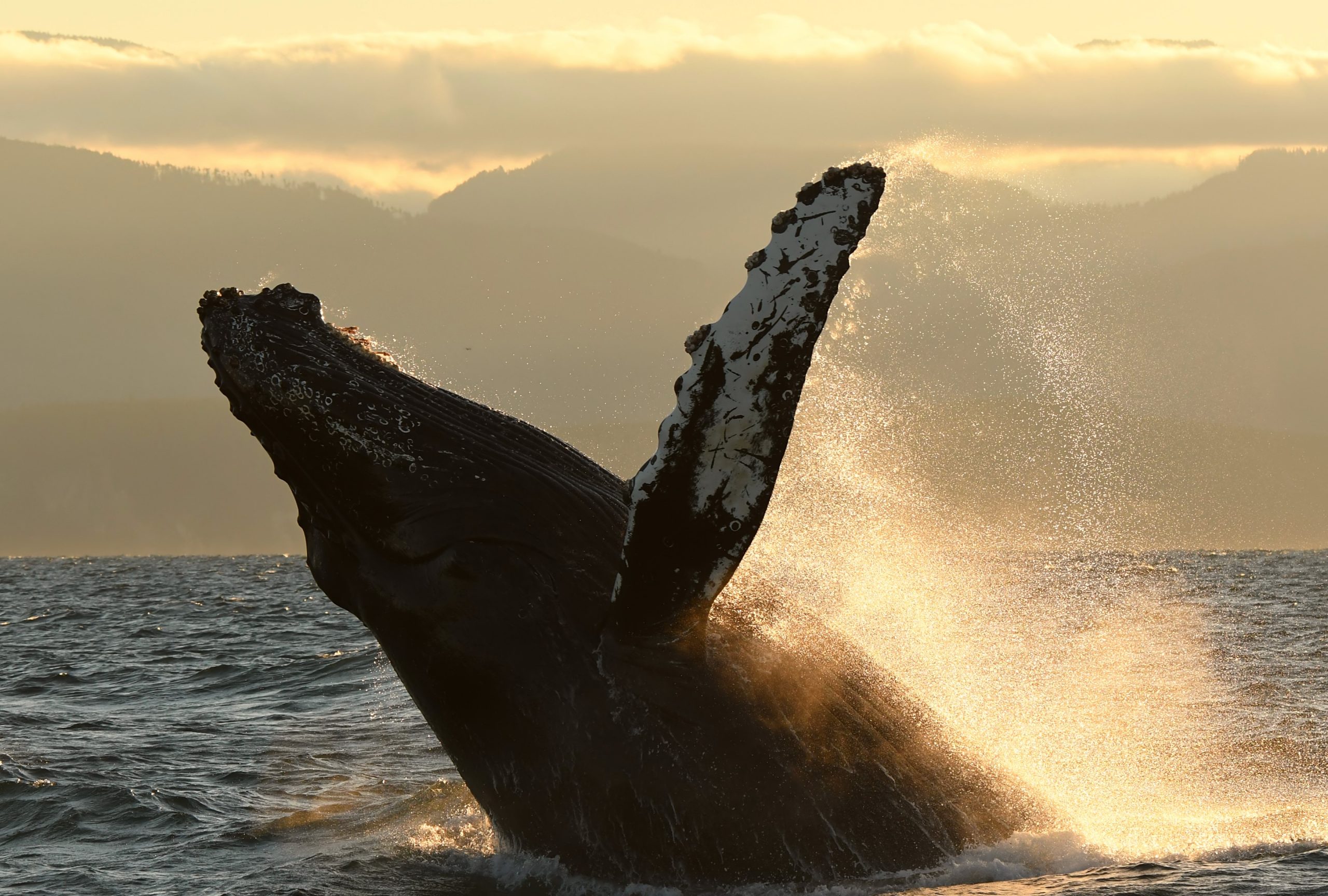In this outdoor, color photograph taken at sea level, we gaze towards the horizon where a massive humpback whale is captured mid-breach. Emerging from the bottom of the frame, the whale’s body is angled up, with its head pointing to the left and its fin thrusting almost straight up, slightly to the right, shedding glistening water droplets. The golden sunlight, streaming from the upper right, casts a radiant glow on the scene, illuminating the whale’s backlit form and highlighting the spray of water it has created. The calm, azure ocean below contrasts with the dramatic, heavy clouds above, tinged with sunlight but hiding the sun itself. The serene sea and sky are subtly colored, reinforcing the focus on the whale's majestic leap. In the distance, faint silhouettes of mountains or foothills add a final touch of grandeur to this striking moment in nature.